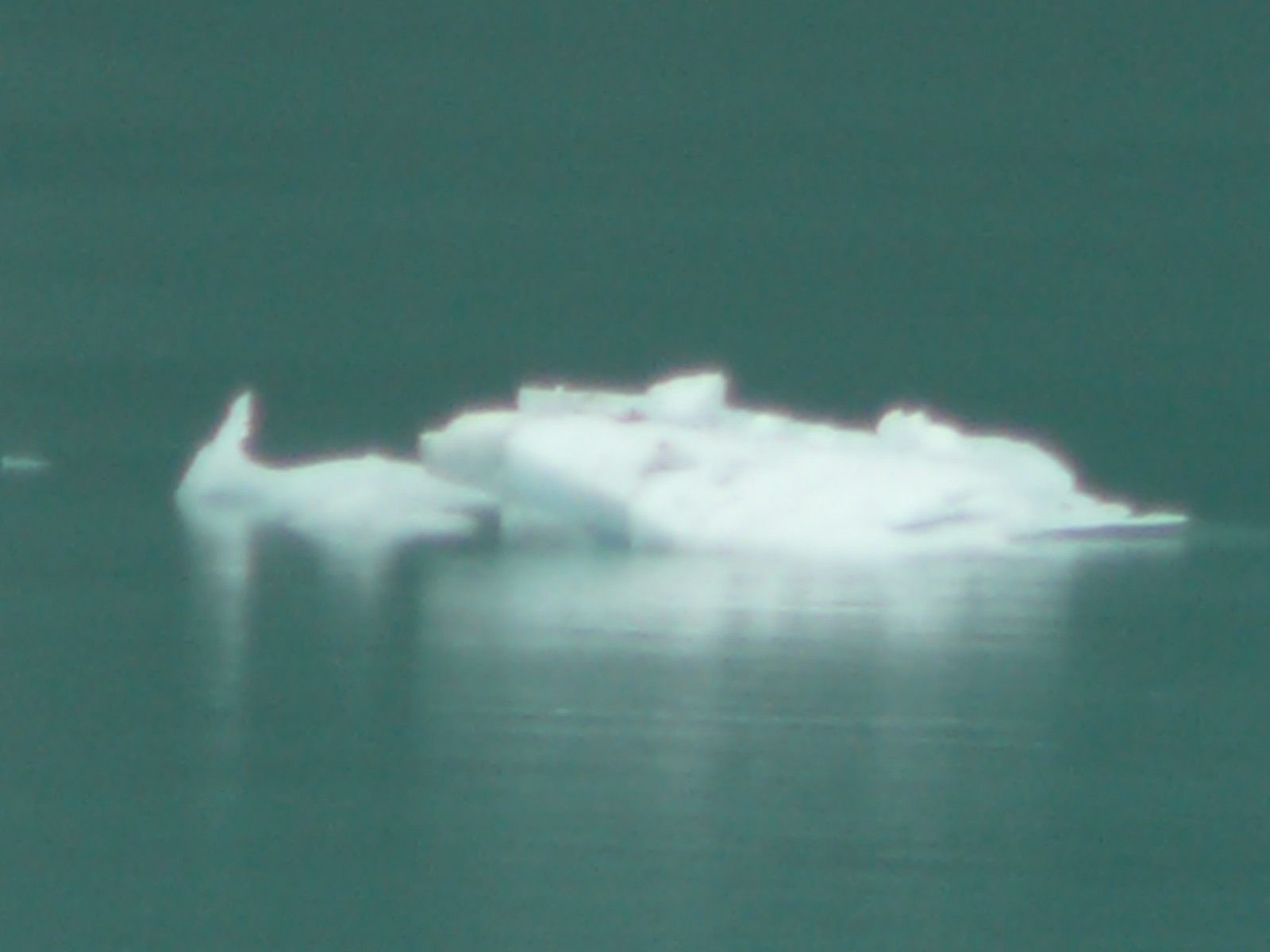The photograph captures a low-quality, grainy, and very blurry black-and-white scene of a body of water with a floating chunk of ice. The image, devoid of clear detail, integrates tones of gray that blend seamlessly, making the horizon nearly indiscernible. The angle suggests the horizon might be positioned around 60% of the image's height, though it's hard to pinpoint as both the water and sky merge into a uniform gray. The central focus is the isolated white chunk of ice, starkly contrasting with the surrounding gray hues, floating in the middle of this nondescript body of water.